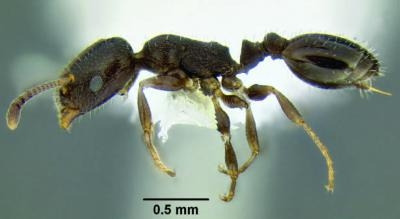The image depicts a black ant positioned sideways, with its head facing to the left. The ant's body is segmented into three distinct parts: the head, thorax, and abdomen. The head, almost charcoal gray, is oval-shaped and features one visible eye and a pair of antennae. The antennae are prominent, emanating out and adding to the ant's meticulous detail. 

The thorax houses five to six segmented legs, which are lengthy and bent in areas, almost as long as the ant itself. The legs extend downward on each side, emphasizing the ant's intricate anatomy. The body is adorned with small, light-colored fine hairs that are predominantly visible towards the rear section but are scattered across the entire body.

The abdomen is a large, oval-shaped segment, nearly spherical, ending in a small spike. The entire body of the ant appears to be encased or suspended, suggesting it might be preserved in a plastic material. Below the foremost leg, there is a horizontal black bar above text that reads "0.5 mm," indicating the scale of measurement. The background is a gradient blend of light blue and white, blurring gently, creating a soft contrast that highlights the ant's detailed features. 

Overall, the image offers a highly magnified and detailed view of the ant, emphasizing its anatomical structure and the fine hairs on its body.